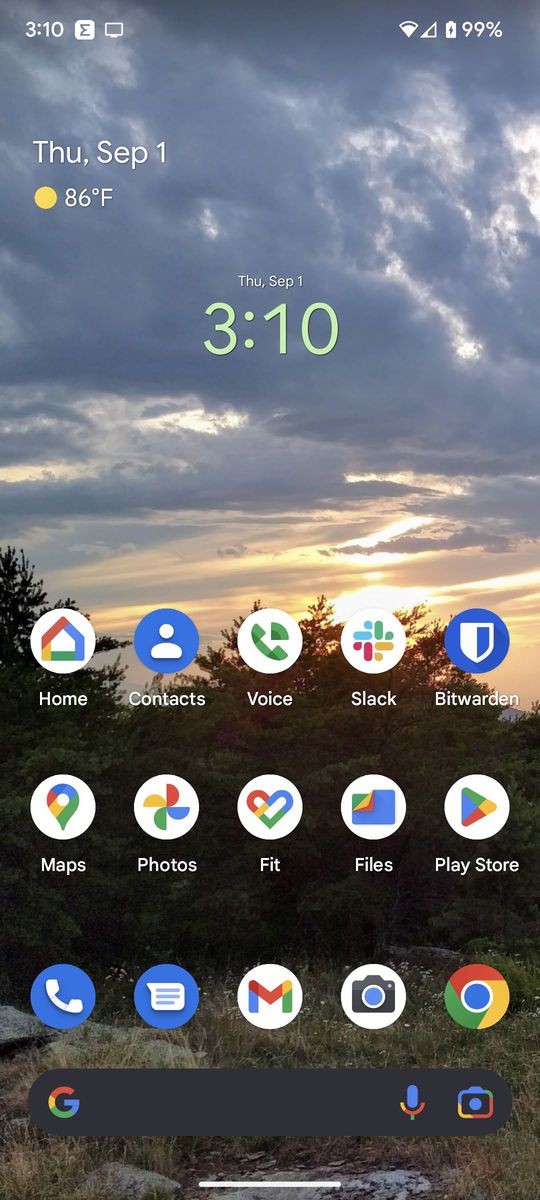**Detailed Caption:**

The image is a screenshot taken from a smartphone's main screen. The wallpaper captures a serene landscape featuring a gray, cloudy sky at the top, transitioning into a warm, yellow-tinged sunset. Beneath, there are trees and bushes, leading down to a visible ground layer, which appears to be covered with grass or rocks.

Overlaying this picturesque background, several standard smartphone indicators can be observed. At the top left corner, the time is displayed, reading "3:10." Opposite this, on the top right, the battery level is shown at 99%, accompanied by the Wi-Fi signal strength icon.

Just below the time, the date is clearly stated as "Thursday, September 1st," and there is a weather indication marked by a yellow dot and a red dot, reporting the temperature as 86°F. 

In the center of the screen, the date "Thursday, September 1st" is reiterated, alongside the time "3:10," which is highlighted in green.

The lower section of the screen is occupied by a grid of app shortcuts, arranged in three rows of five circles each, totaling 15 icons. Among these, notable icons include:
- A white circle featuring a vibrant, rainbow-colored home icon with the label "Home" written in white.
- A blue circle with a white person icon, labeled "Contacts."
- A white circle containing a green telephone icon, titled "Voice."
- Additionally, there are icons for the camera, the Google Chrome browser (depicted as a multicolored, swirling circle), and more.

At the very bottom lies a search bar, which is black with a "G" for Google on the left. To the right of this search bar, there are colorful icons for a microphone and a camera, indicating Google voice search and Google Lens functionalities.